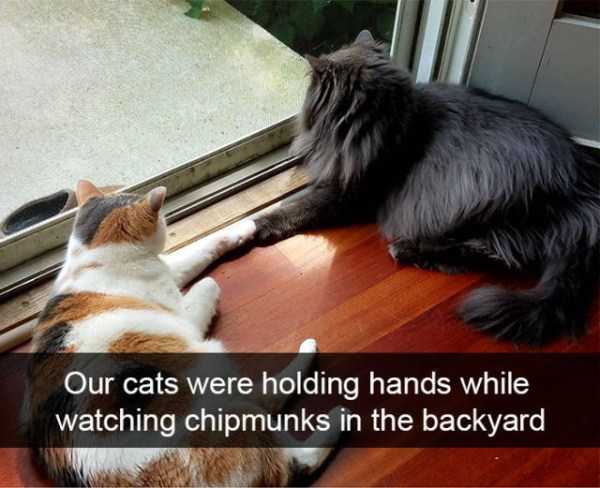In this photograph, two domestic cats, a black long-haired cat on the right and a calico short-haired cat on the left, are laying on a glossy hardwood floor inside a house. They are both gazing out through a white-framed screen door. Their front left paws touch, appearing as if they are holding hands while watching the backyard. The calico, featuring white, black, and orange fur, lies closer to the left side of the frame. The black cat, with plush fur, is seen on all fours to the right. Outside the screen door, there is a concrete slab and a moccasin shoe visible. The caption in front of the image, enclosed in an opaque black box with white font, reads, "Our cats were holding hands while watching chipmunks in the backyard," indicating that it was likely intended as a social media post. The scene takes place during the day in the spring or summer, as suggested by the visible greenery.